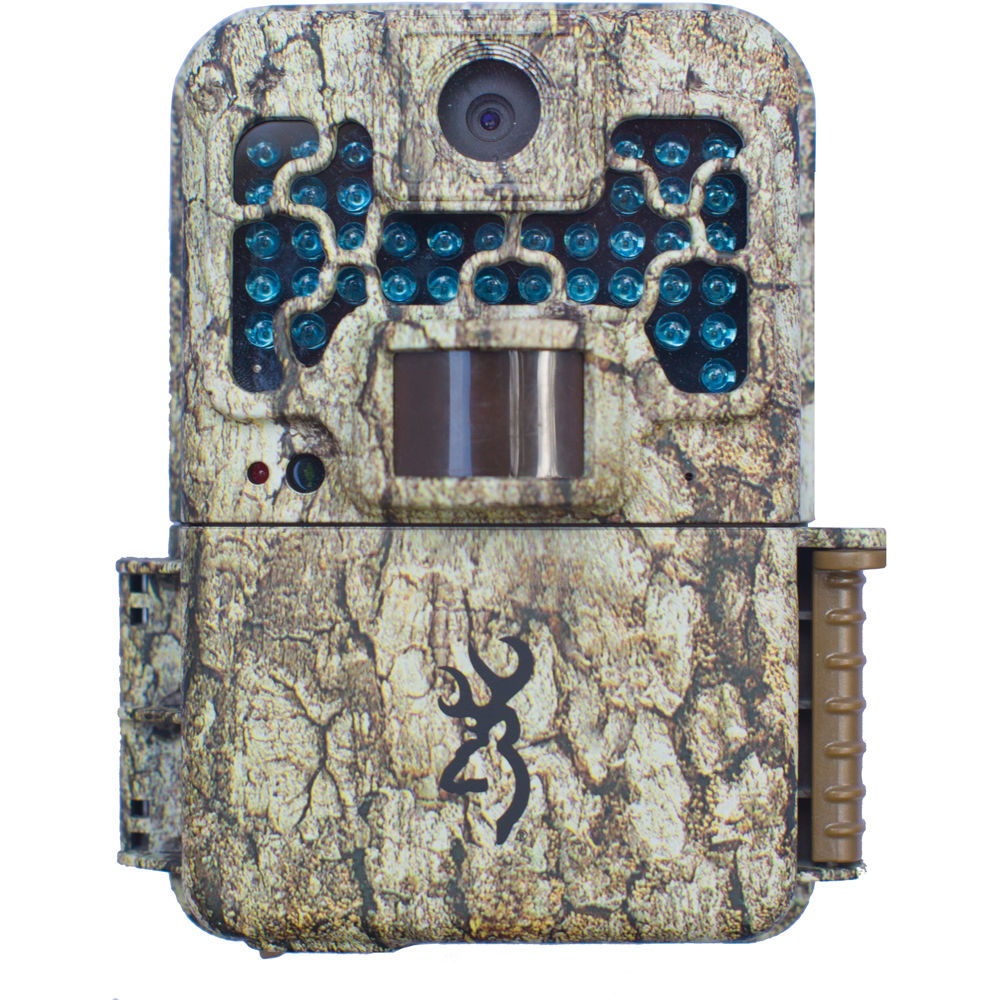This highly detailed photographic image features a vertical rectangular object against a white background, resembling a trail camera encased in a plastic box. The object has rounded edges and appears to have a bark-like camouflage pattern in hues of gray with darker cracks, giving it a stone-like appearance, and brown markings.

At the top of the object is a prominent round hole housing a camera lens, surrounded by indented square pieces with a recessed blue dot in the center. The upper portion of the rectangle has a horizontal cut-out area with various light blue LED-type lights arranged both vertically and horizontally, resembling a white 'H' framed by gray strands connecting to the outer edges.

Suspended from the central hole is a polished gray or silver metal cylinder with a brown handle.

The lower portion of the object features another noticeable division, displaying a distinct symbol that resembles an Arabic or stylized 'X' in black, characterized by curvy prongs. The bottom left segment has a rusty hinge next to square holes, while the bottom right displays a short cylindrical pin with ridged notches that connect to a brown plastic piece.

Overall, the image does not include any readable text, and the setting remains undefined beyond the stark, solid white background.